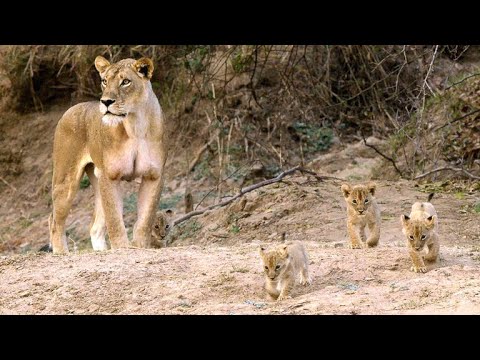In this daytime photograph set in a desert-like terrain, a vigilant mother lion stands to the left of the frame, her alert gaze fixed off screen. The earth beneath is a light brown, sandy hue, with sparse, leafless foliage and sticks in the background, along with a few green shrubs scattered around. Nestled under her left leg is a cub, appearing to seek the mother’s protection, while displaying a mix of golden, brown, tan, and white fur. The belly and breast areas of the lions are notably light in color, with some of the cubs showing hints of white and gray at their centers.

In front of the lioness, three additional cubs are advancing towards the viewer. The cub on the left is the furthest ahead, the one on the right is crouched and near the center, and the middle cub trails slightly behind. All the cubs share a similar coloration to their mother, featuring a blend of orangish-brown top sides and lighter, beige, and white undersides. Some of the cubs also sport dark spots on their heads and snouts. The scene embodies a moment of family unity and watchfulness amidst a raw, arid landscape.